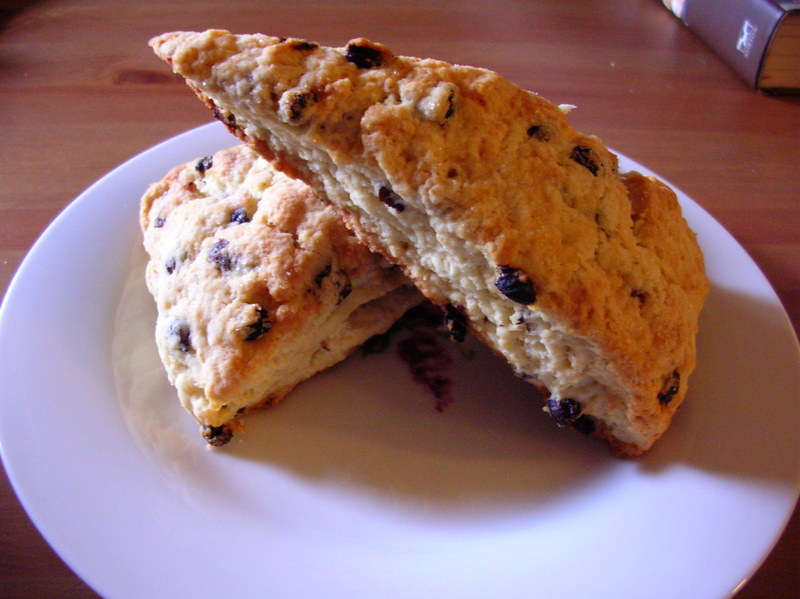The image features two triangular, fluffy pastries, which appear to be blueberry scones, resting on a smooth, white plate. The golden-brown exterior of the scones is complemented by their off-white, flaky interior, with small, dark blueberry pieces nestled throughout. One scone lies flat while the other is propped up at a 45-degree angle, showcasing its crumbly texture. This arrangement sits on a light pink and tan-colored wooden tabletop, bathed in soft sunlight. In the upper right corner of the image, the spine of a thick, brown hardcover book with a white logo is visible, adding a touch of homely charm to the scene.